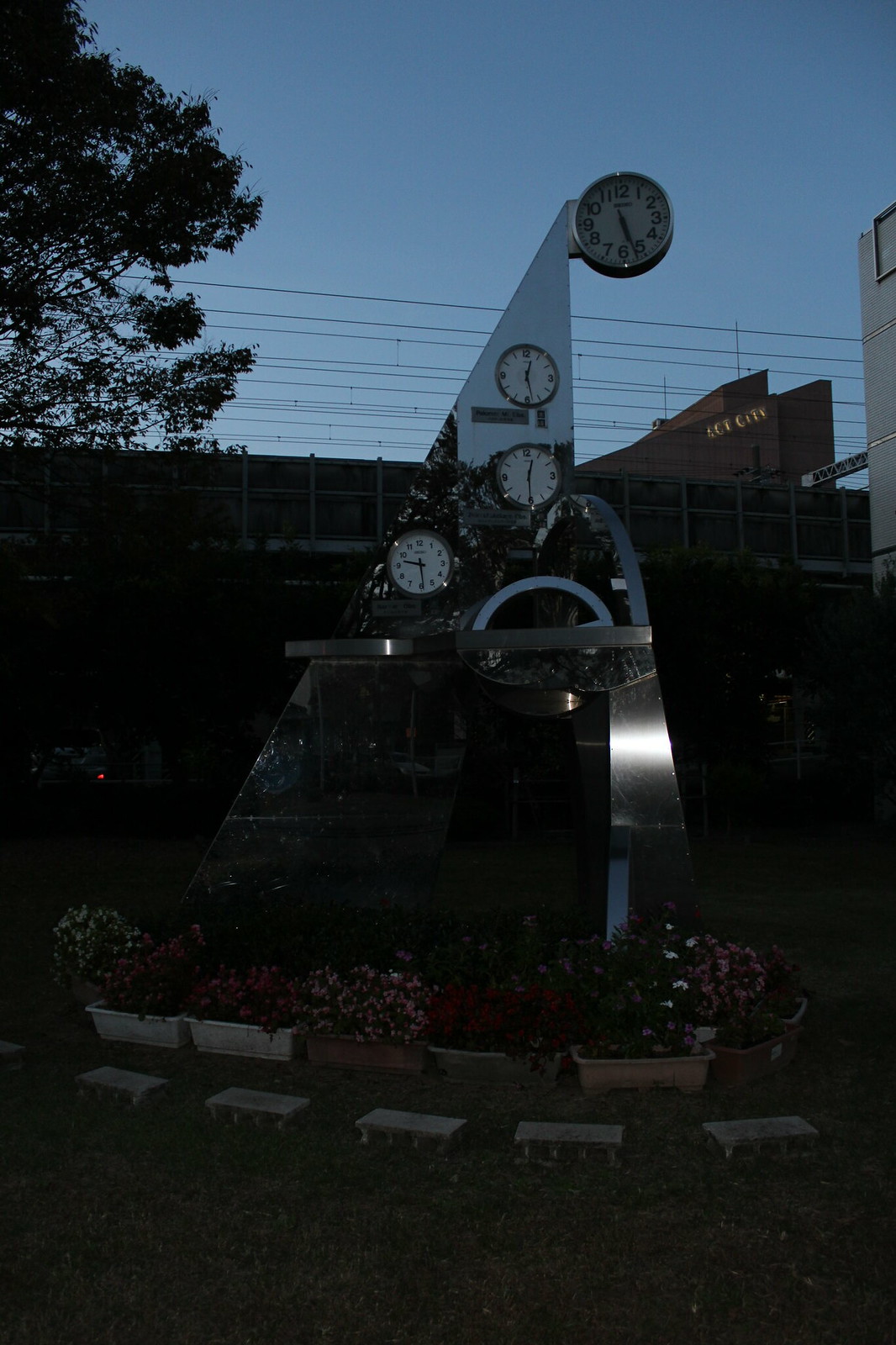In this rectangular photograph, we observe a scene captured in what appears to be the later part of the day. The sky remains a clear blue, but substantial portions of the area are shrouded in shadows. Dominating the image is an overpass positioned above our line of sight, surrounded by a series of wires that seem to act as railing.

Beneath the overpass and prominently placed in the foreground is a striking triangular sculpture. This unique piece seems to be constructed primarily from wire and metal materials, with elements that suggest it may be crafted from copper or brass. At its base, the material appears woven in a wire formation, leading upwards to a pointed tip.

Embedded within the triangular structure are three distinct white-faced clocks, each displaying different times. The topmost clock reads 12:27, positioned centrally a second clock shows 12:30, and at the bottom left, a third clock indicates 9:29. Attached off to the right side of the sculpture, though still part of the structure, is a larger clock. This additional timepiece features numeric numbers from 1 to 12 and displays the time as 5:27 with its black hands.

The combination of the architectural elements and the public art installation offers a complex interplay of form, function, and time, grounded against the shaded urban landscape.